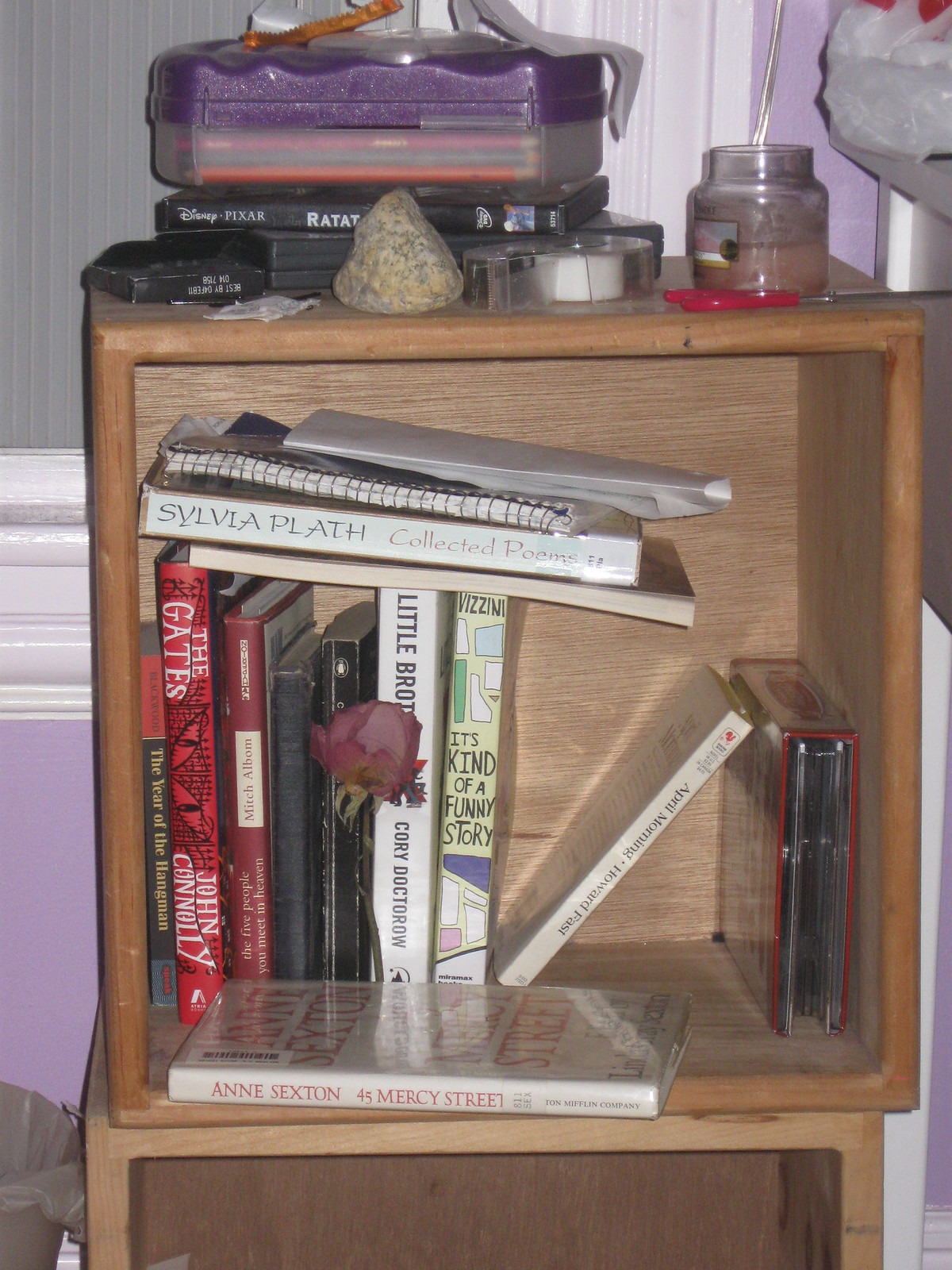The photograph depicts a cluttered wooden shelf situated inside a room with medium, regular lighting. The background showcases a gray wall adorned with vertical lines, a white trim, and light purple paint below it, creating a visually interesting contrast. This wooden shelf, which appears to be part of a stacked unit, reveals a middle section filled with various books, maps, and papers haphazardly placed atop one another. Visible titles include *45 Mercy Street* by Anne Sexton, *Collected Poems* by Sylvia Plath, *It's Kind of a Funny Story* by Ned Vizzini, *April Morning* by Howard Fast, *The Gates* by John Connolly, *The Year of the Hangman* by Gary Blackwood, and *The Five People You Meet in Heaven* by Mitch Albom. The shelf is topped with an assortment of items, including a rock, scissors, tape, a candle, a pencil box filled with colored pencils, a Disney movie DVD, some trash, gum, and stencils, encapsulating a mix of arts and crafts materials and sundry items. The wooden shelf rests on top of another wooden box, which is only partially visible in the image.